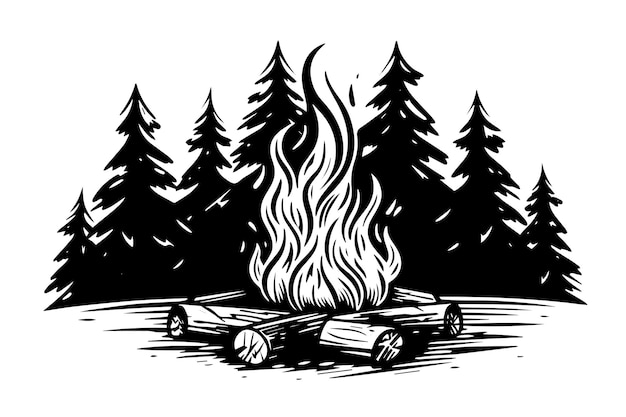In this detailed black-and-white pencil illustration, a vividly drawn campfire takes center stage. The campfire consists of five logs arranged beneath moderately high flames, which are depicted with intricate black lines and white highlights to accentuate their shape and movement. Surrounding the fire are sketches representing the ground, adding to the rustic ambiance of the scene. The background features a dense forest of seven large pine trees, meticulously illustrated in dark black with white highlights, as if subtly illuminated by the campfire's glow. The pine trees, with their detailed branches, dominate the horizon and stretch across the entire width of the picture, evoking a tranquil, nighttime setting. Despite the absence of text or human figures, the quality and details of the drawing vividly capture the essence of an outdoor campfire in the woods.